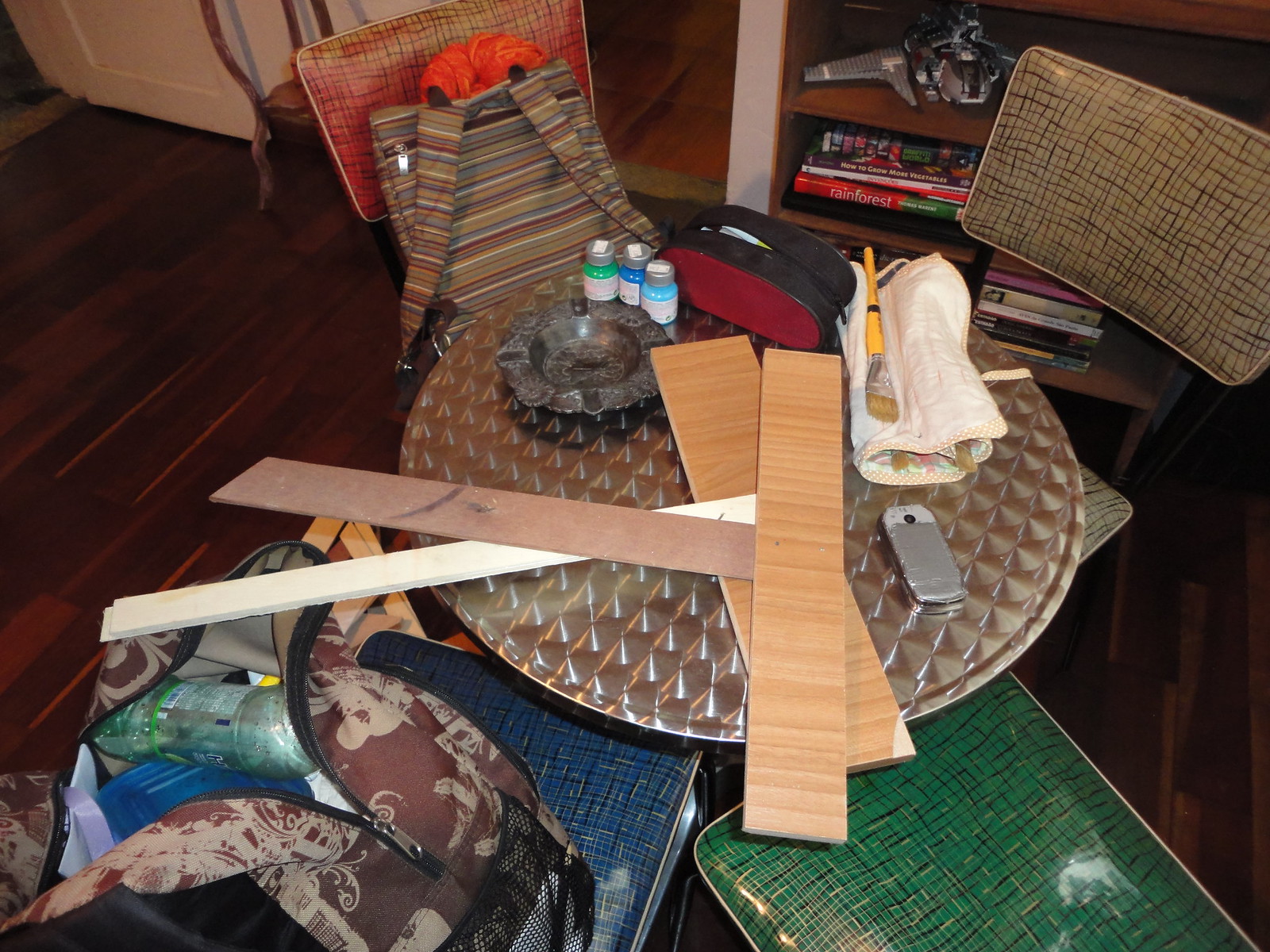The image captures a meticulously detailed section of a living room. A small, circular, flat table sits at the center, surrounded by four chairs. The chair in the bottom left corner is adorned with a blue square cushion, atop which rests a brown and black backpack with its zipper open, revealing an empty green bottle and a blue object inside. To its right, only the green square cushion of another chair is visible. 

The table, brown and round, is strewn with various items: several planks of wood in different shades (two light brown, one dark brown, and one white), the backside of a mostly gray with white cell phone, a white towel paired with a yellow paintbrush, three small bottles, a black object with a red front, and an ashtray. 

In the background, a chair with a red back is visible, next to a striped backpack topped with an orange object. Part of a lower bookshelf is seen in the back right, while the flooring throughout the room is a dark brown, contrasting with the underside of a white wall visible in the upper left corner.